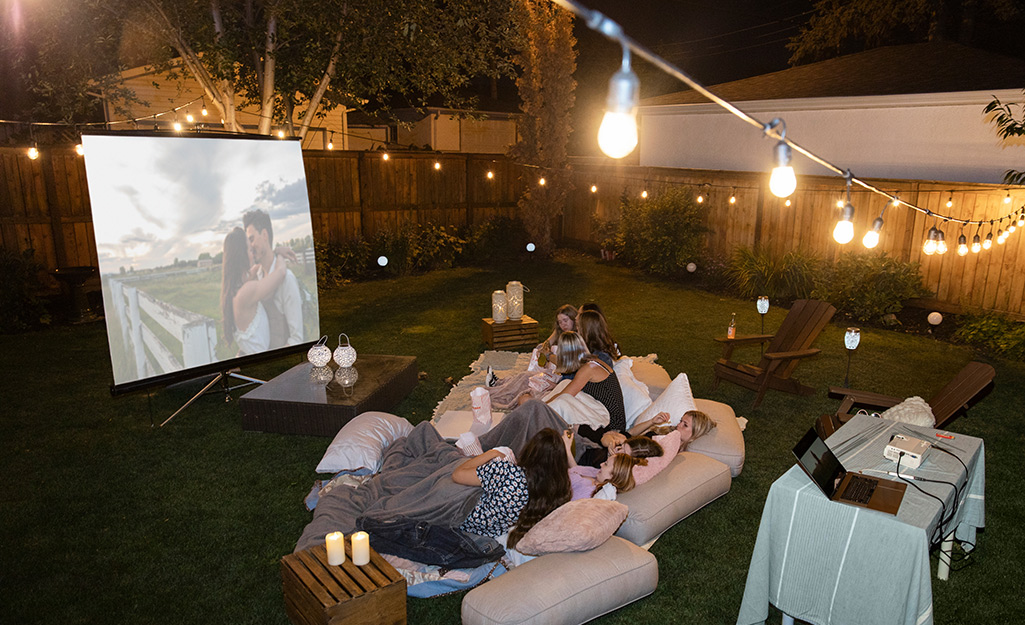The image captures a cozy nighttime scene in a backyard surrounded by a wooden fence and illuminated with medium-sized string lights. The central focus is an outdoor movie screening, where a group of about eight or nine young women are watching a romantic movie projected onto a large 10 by 10-foot screen. The screen displays a couple embracing next to a white fence in a sunlit setting. The backyard setup includes several comfortable reclining areas made of beige cushions, white pillows, gray blankets, and couch cushions arranged on the grass. In addition to the seating area, there's a table with a light-colored or bluish tablecloth behind the girls, holding a white projector and a laptop. The cozy ambiance is enhanced by the presence of candles placed in crates, adding a warm glow to the space. The lawn features a few lawn chairs, and the surroundings include other houses visible beyond the wooden fence. The scene exudes a laid-back, communal vibe, suggesting a sleepover or casual gathering under the stars.